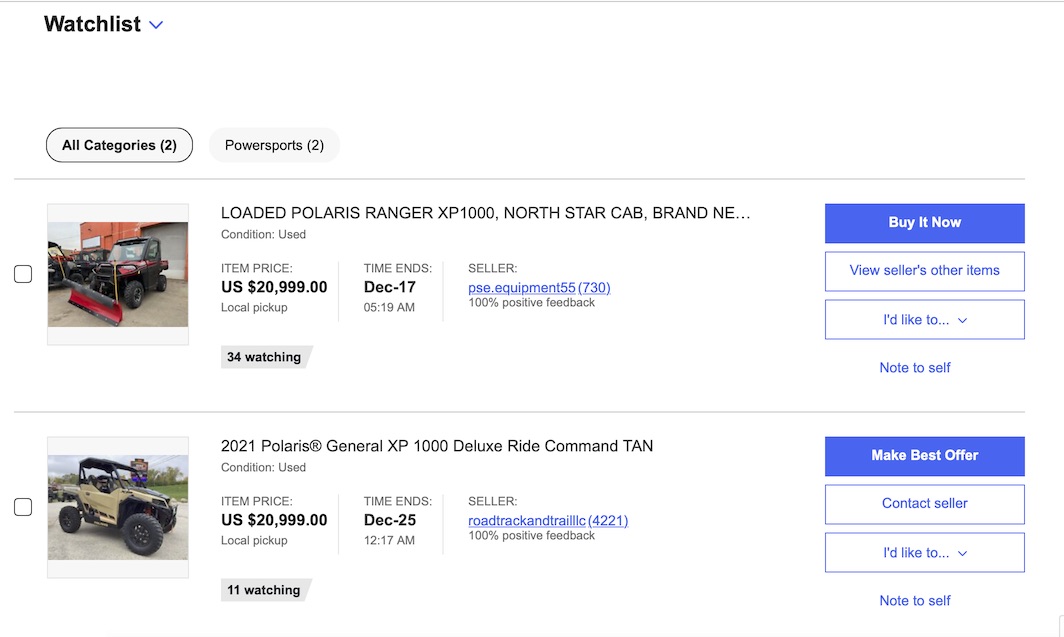At the top of the image, there is a navigation bar with a horizontal line stretching from left to right. Just below this line, in bold black letters, "Watch List" is prominently displayed. Directly next to "Watch List" is a drop-down button. Beneath that, the text "All Categories" can be seen alongside another button labeled "Power Sports."

Central to the image is a picture of a machinery item—a snowplow-equipped vehicle identified as a "Loaded Polaris Ranger XP 1000 Northstar Cab." The vehicle is described as being in "brand-new condition." This used item is listed at a price of US $20,999, and it is available for local pickup in Washington. The listing’s timestamp reads December 17, 05:19 a.m. The seller is identified as "PSE Equipment," boasting a 100% positive feedback rating with 55 reviews.

Below this, there is another listing for a "2021 Polaris General XP 1000 Deluxe Ride Command," in "TAN" color. This vehicle is also noted as a used item with a price of US $20,999. The listing’s timestamp for this item is December 25, 12:17 a.m.